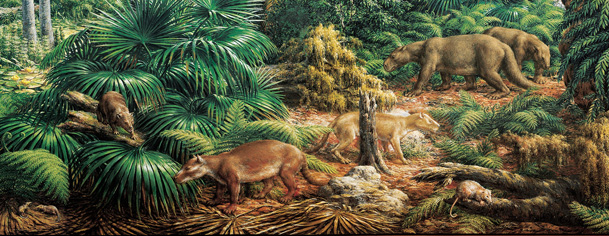The image is a detailed pencil and color drawing of a prehistoric jungle teeming with various unusual mammals. Dominating the composition is a dense array of foliage, including small, fan-like palm trees, overgrown ferns, and tree trunks adorned with green lichen. In the top right corner, a large muscly creature with thick brown fur and a horse-like head strides on four legs, its imposing form hinting at its dominance. Below, in the bottom right corner, a smaller, white and tan creature with a pointed nose, resembling a modern-day possum, surveys its surroundings cautiously. The middle of the scene features several tapir-like animals with brown fur, characterized by their long, wide, and pointed tails. These creatures vary in size, and their interactions hint at a rich ecosystem. One particular tapir-like animal, resembling a tiger in its tan color, stands before a broken tree stump, facing the viewer with an alert expression. The left side of the scene is filled with stacked palm leaves and an animal perched atop them, creating a sense of depth and intricate layering. Overall, the horizontally oriented drawing vividly captures the vibrancy and complexity of the prehistoric jungle.